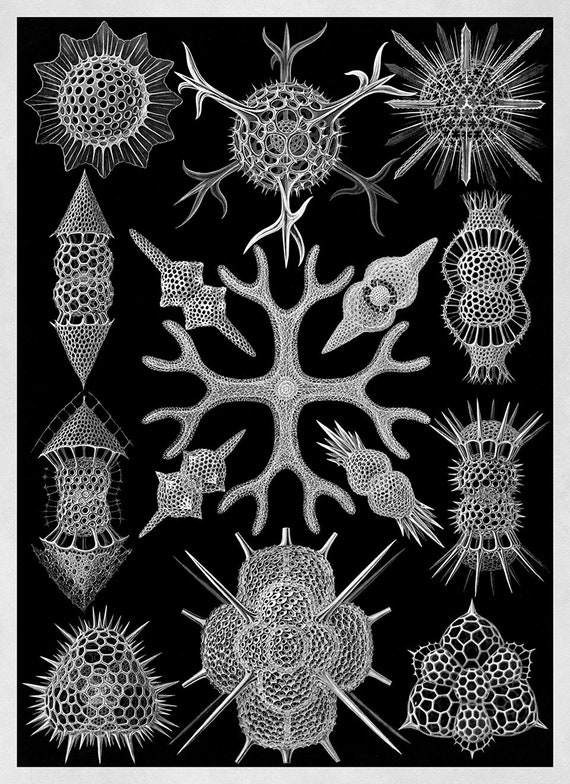The black and white image features a striking contrast with a black background and intricate white outlines of various geometric structures, resembling single-celled organisms or abstract representations of bacteria. There are about a dozen distinct shapes, many of which have a honeycomb-like appearance with multiple holes and protrusions. Central to the composition is a cross-like structure surrounded by four other similar forms. The uppermost shape has a sunburst pattern emanating from a honeycomb center, while another prominent figure below it features a triangular base with honeycomb details. The arrangement follows a symmetrical pattern: three shapes at the top, three at the bottom, and four on each side, totaling around ten peripheral objects. The image lacks any text and is framed by a white or gray outline, enhancing its abstract, almost scientific aesthetic.